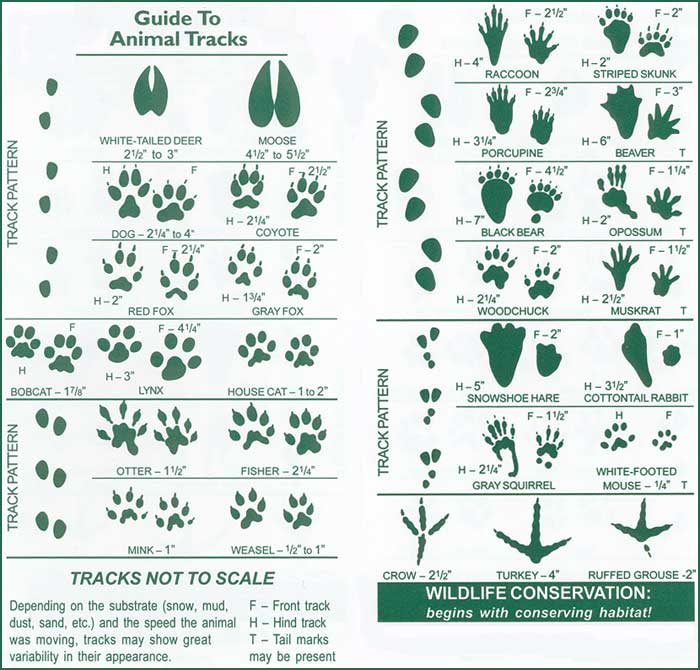This detailed guide to animal tracks, printed on white paper with dark green text, appears designed for use in wildlife centers, national parks, or state parks. It comprehensively displays a range of animal tracks alongside patterns and dimensions (presented in inches but with a note that tracks are not to scale) for various species such as white-tailed deer, moose, dog, coyote, red fox, gray fox, bobcat, lynx, house cat, otter, fisher, mink, and weasel. The diagram also extends further, featuring additional tracks on the right-hand side for animals like porcupines, beavers, squirrels, geese, raccoons, striped skunks, black bears, opossums, woodchucks, muskrats, snowshoe hares, cottontail rabbits, gray squirrels, white-footed mice, crows, turkeys, and ruffed grouses. With detailed illustrations of each animal's gaits and a bottom banner that emphasizes "wildlife conservation begins with conserving habitat," this guide serves as a detailed educational tool, with helpful annotations such as "F" for front track, "H" for hind track, and "T" for tail marks that may be present.